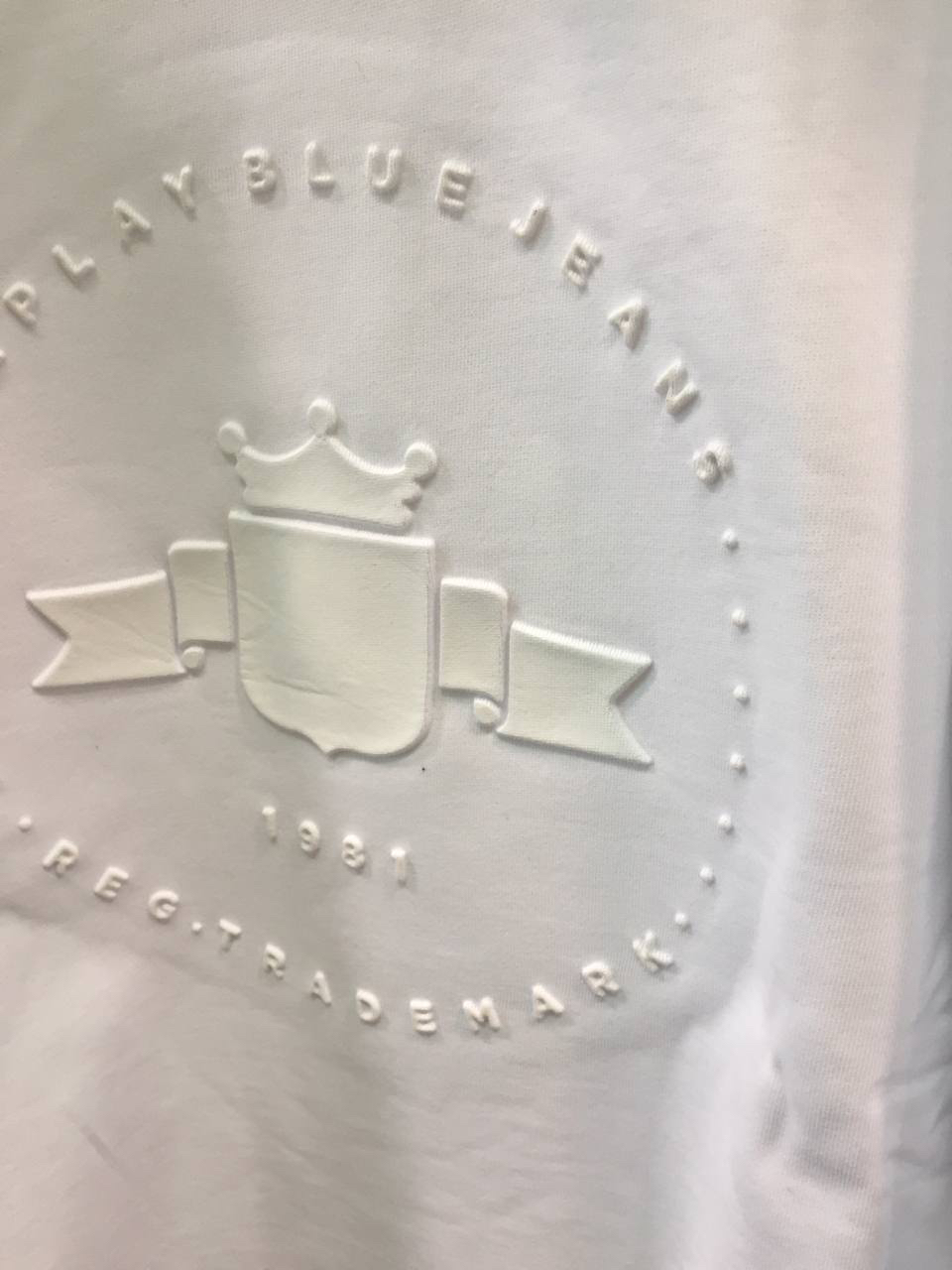The image is a close-up of a piece of white fabric or cloth, possibly part of a piece of clothing or a tote bag. Central to the fabric is a rubbery, embossed emblem, also in a white or cream color. This emblem features a shield-like shape with ribbons on either side and a simple crown with three points and small circles on top. At the center of the emblem, beneath the crown, is the text "1981." Encircling the shield are raised dots on the left and right sides, with the top of the circle reading "Play Blue Jeans" and the bottom stating "Reg Trademark." The fabric appears to have been crumpled at some point and then smoothed out.